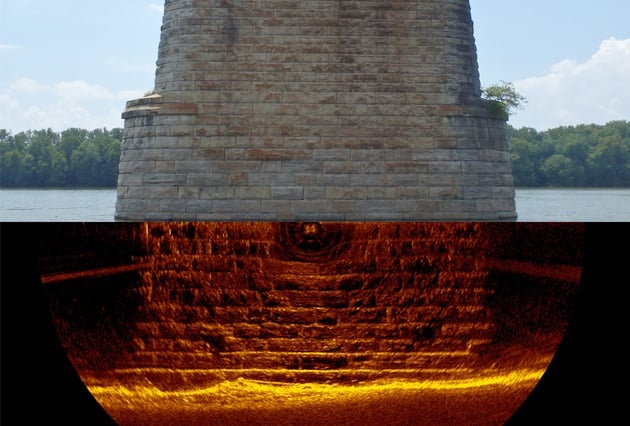The image presents a split visual, divided into an upper and a lower half, each with distinct yet connected elements. The top half features a realistic photograph of a brick structure with a vaguely triangular shape, appearing almost cylindrical, possibly a support pillar for a bridge. The bricks range in color from gray to beige to almost red. Surrounding this structure is a calm, pale blue body of water, a rich, lush green tree line, and a sky filled with fluffy white clouds. Some vegetation is growing alongside the right side of the brick structure.

The bottom half of the image contrasts sharply, depicting what seems to be an underground dungeon. The same brick material as the top structure continues here, but the scene is bathed in an ominous red and orange glow, suggesting heat or fire. The background is predominantly black, emphasizing the fiery highlights, and the composition of the lower half is cropped into a semicircle. Together, the two halves create a juxtaposition of serene and intense atmospheres, with no text present in the image to provide further context.